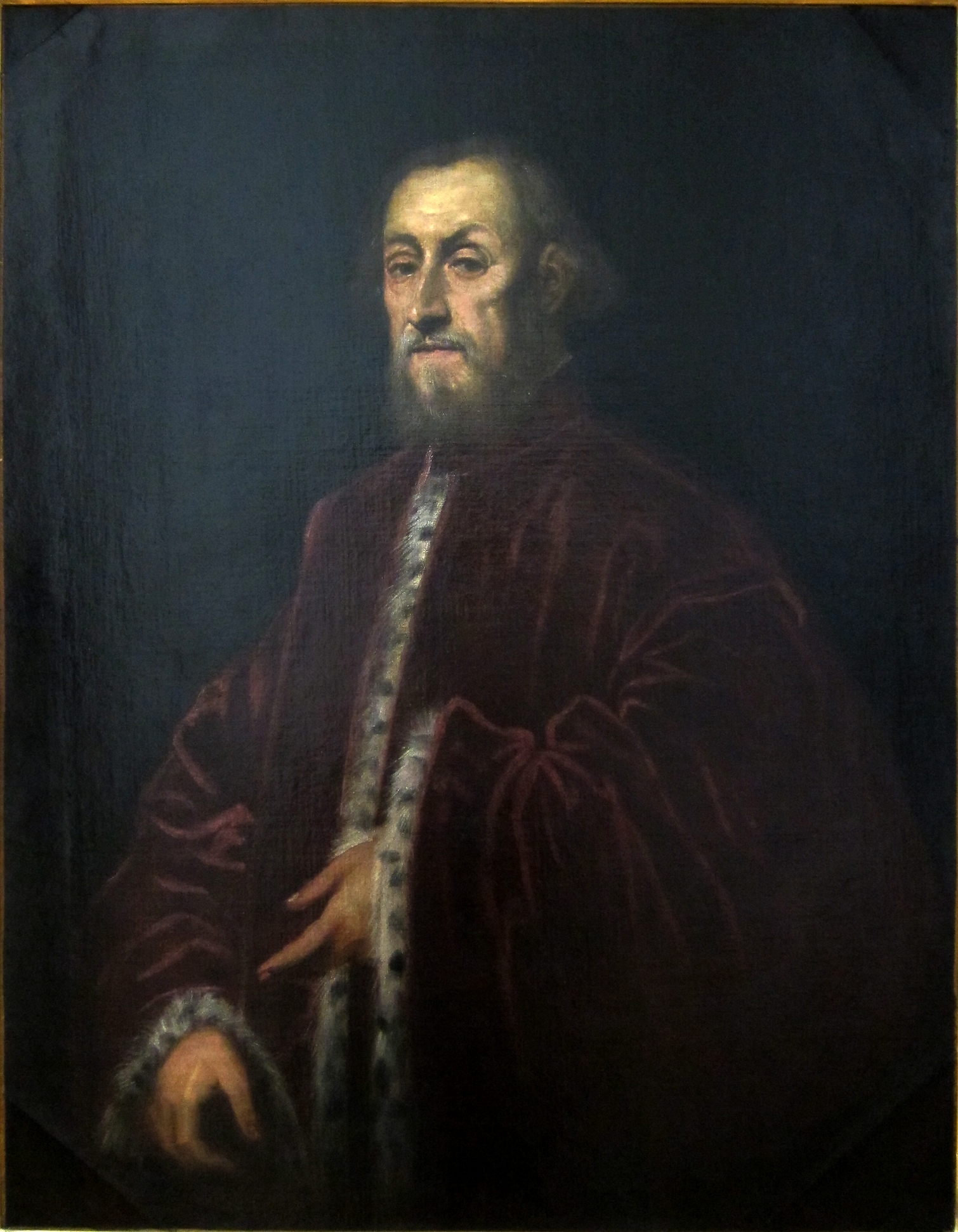The image is a classical portrait painting of an older Caucasian man, likely in his 60s or 70s, set against a dark black background. He is dressed in a deep, almost black, velvet robe with a rich dark red or purple hue. The robe features distinctive white and black spotted fur trim around the cuffs and down the front. The man has a scruffy gray beard and mustache with longish hair down to his collar, noticeably balding on top. His expression is contemplative as he grasps the tip of a cane with one hand, while his finger on the other hand points downward. The left side of the image is subtly lighter, perhaps suggesting sunlight streaming in, though the background and robe blend into each other due to their dark tones. The overall attire suggests the painting likely dates from the medieval period.